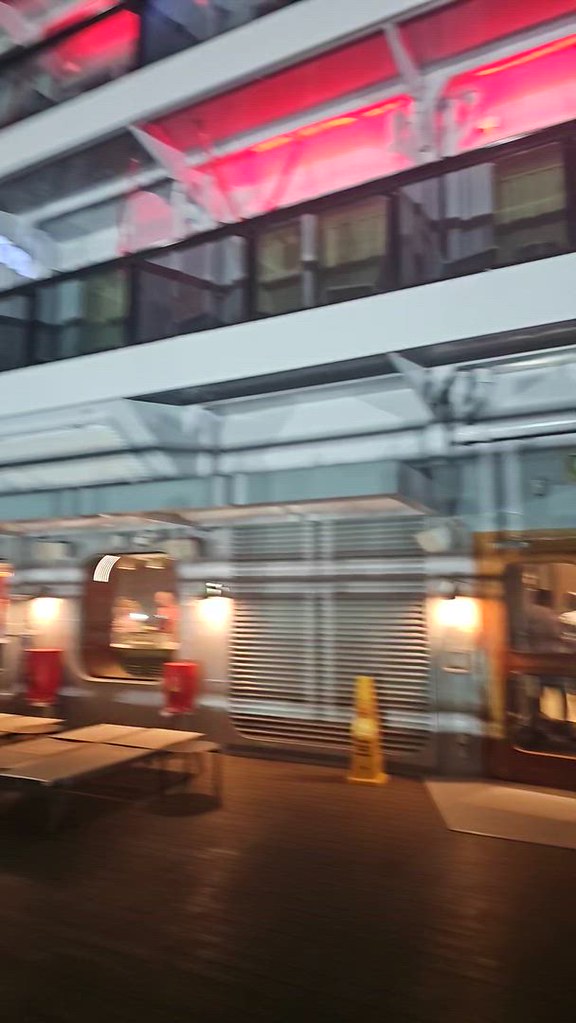This vertically oriented rectangular photograph captures the interior of what could be a hotel courtyard or perhaps more likely the inside of a cruise ship. The image is framed from an elevated vantage point, overlooking a black balcony with clear glass panels. Beyond the balcony, tall white windows stretch up to the ceiling, interspersed with a few brown doors, adding a contrasting element. 

On the lower level that is also visible, several tables are accompanied by low bar stool-style seats, arranged on a glistening brown floor that catches the light. The walls are painted in a pristine white with accents of light blue, lending a clean and airy feel to the space. Elegant portal windows punctuate the lower floor, adding a nautical touch to the refined setting.